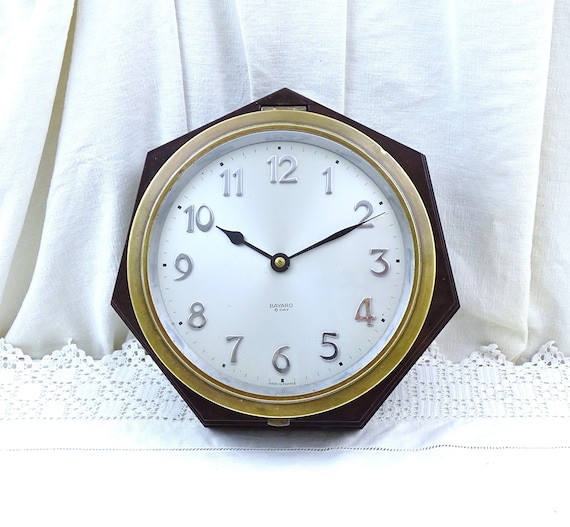This image depicts a traditionally designed clock, featuring a white face with silver numbers and black hands, one for the hour and one for the minute. The clock’s center is surrounded by a gold circular ring. Encasing this ring is a seven-sided black frame, though one person suggested it might be dark brown and possibly wooden, albeit with no visible wood grain. The clock is propped against a white curtain, atop a delicately patterned white lace doily. The hem of the doily or lace has a subtle checkerboard pattern with squares and tiny holes. The clock's hands are positioned such that it reads around 10:02 or 10:03. There's also a logo or name on the clock face, possibly reading "Bayard," but it's too small to discern clearly. This staged setup evokes a vintage or old-fashioned aesthetic, similar to what one might find in a grandparent's home.